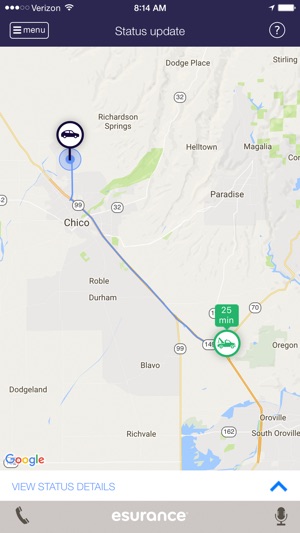The image is a screenshot from a mobile app user interface. At the top center, it displays the time as 8:14 AM. The top right corner shows a full battery icon, and the upper left corner indicates a Verizon service with 3 out of 5 bars and full Wi-Fi connectivity. Just below the time, the title "Status Update" is prominently displayed. To the left of this title, there is a menu button, and to the right, a question mark button.

Dominating most of the screen is a map, featuring various navigation details. A green car icon, possibly representing a vehicle equipped with a crane or a tow truck, is marked on the map. Above this icon, the text reads "25 minutes." The car icon is connected to a location marker, identified by a black circle containing a normal car illustration, situated near Chico. A small Google logo resides in the bottom left corner of the map.

At the bottom segment of the screenshot, the text "View Status Details" is clearly visible, with "Insurance" labeled in the center. Additionally, a call button is positioned in the bottom left corner, and a microphone button is located in the bottom right corner of the interface.